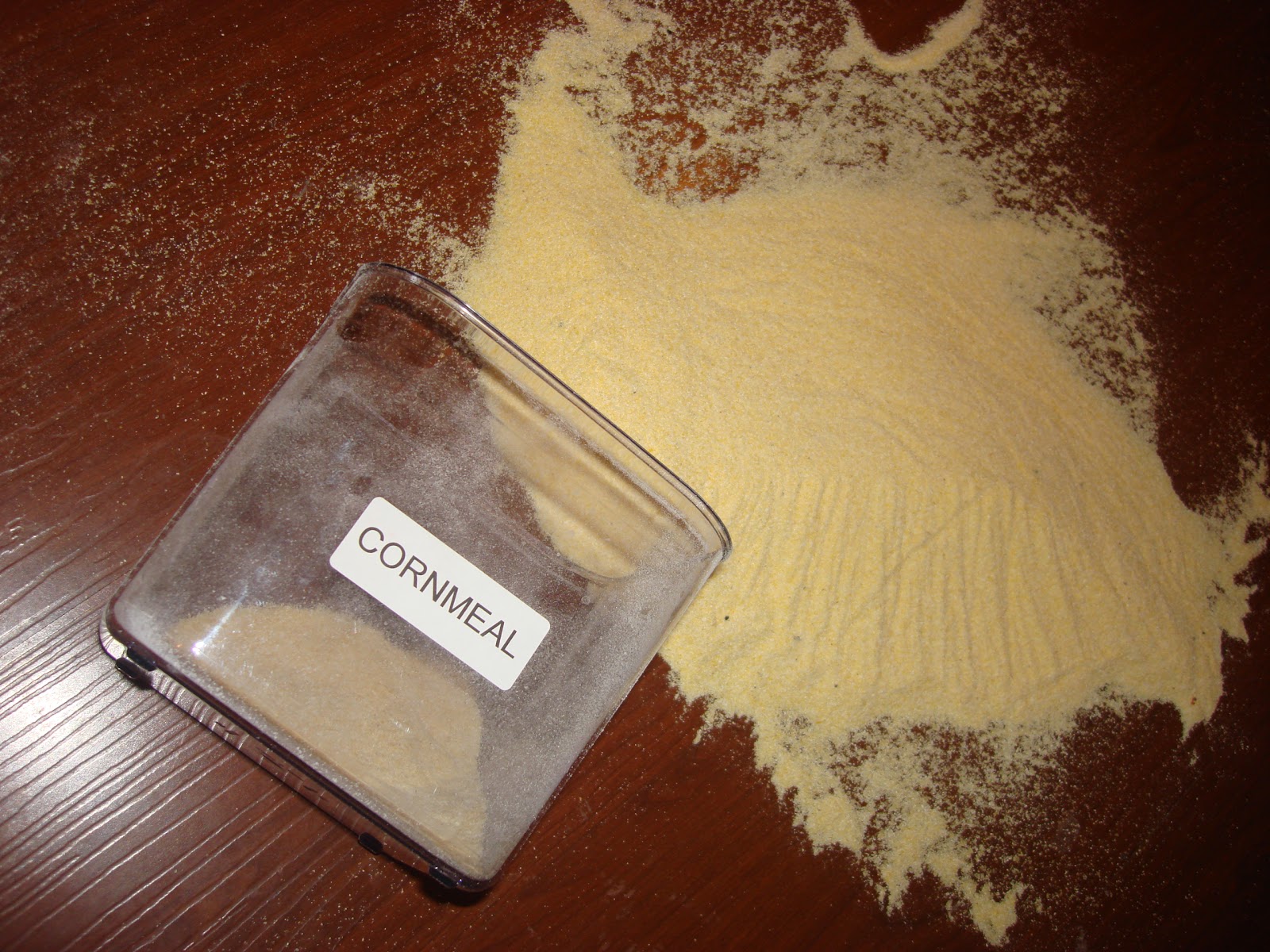The image depicts a clear plastic container without a lid, labeled "CORNMEAL" in all caps black text on a white label. The container, which has only a small amount of cornmeal left inside, has been tipped over, causing the majority of its contents to spill onto a reddish-brown surface that could be a table or floor. The cornmeal is scattered extensively across the surface, with most of it concentrated in the upper right-hand side and the middle of the image. Some of the cornmeal appears to have been brushed into specific spots, creating an inverted arc and a small pile, indicating a possible attempt to start cleaning up. Despite this, the bulk of the cornmeal remains spread out, reaching even into the lower right and upper left corners of the image. The rich brown surface adds a lush and polished look to the scene, but there is no further context or explanation provided for the spill.